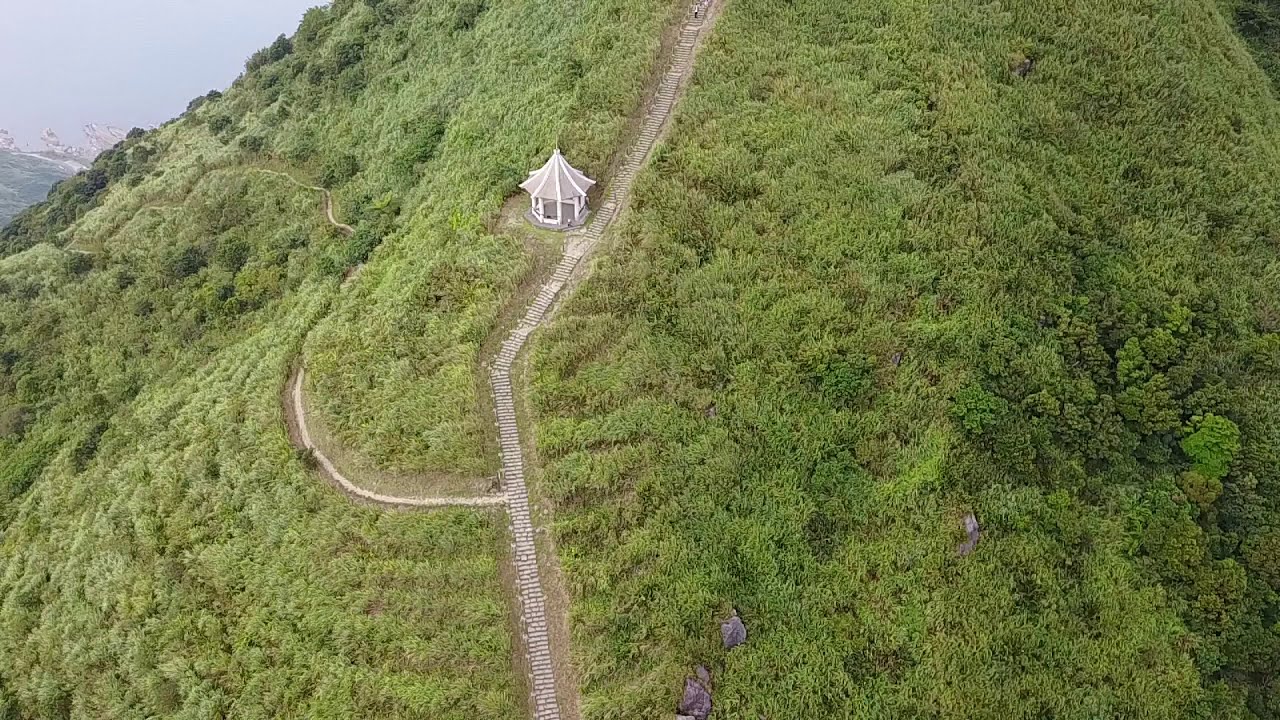This aerial photograph captures a lush, grassy mountaintop, featuring a prominent ridge adorned with a stone pathway that ascends its side. Central to this picturesque scene is a white, gazebo-like structure that resembles an Asian pagoda, positioned roughly halfway up the path. The pathway, crafted from wooden planks with white boards and surrounded by patches of dirt, extends up the hill with an offshoot veering to the left, hinted at by a well-trodden path through dense clusters of trees. The vibrant greenery of the hillside is sporadically interrupted by rocks, adding to its rugged charm. In the upper left corner, beyond the descending hill, a hazy glimpse of what appears to be the ocean is visible, alongside distant, snow-capped mountains beneath a blue sky, completing this serene landscape.